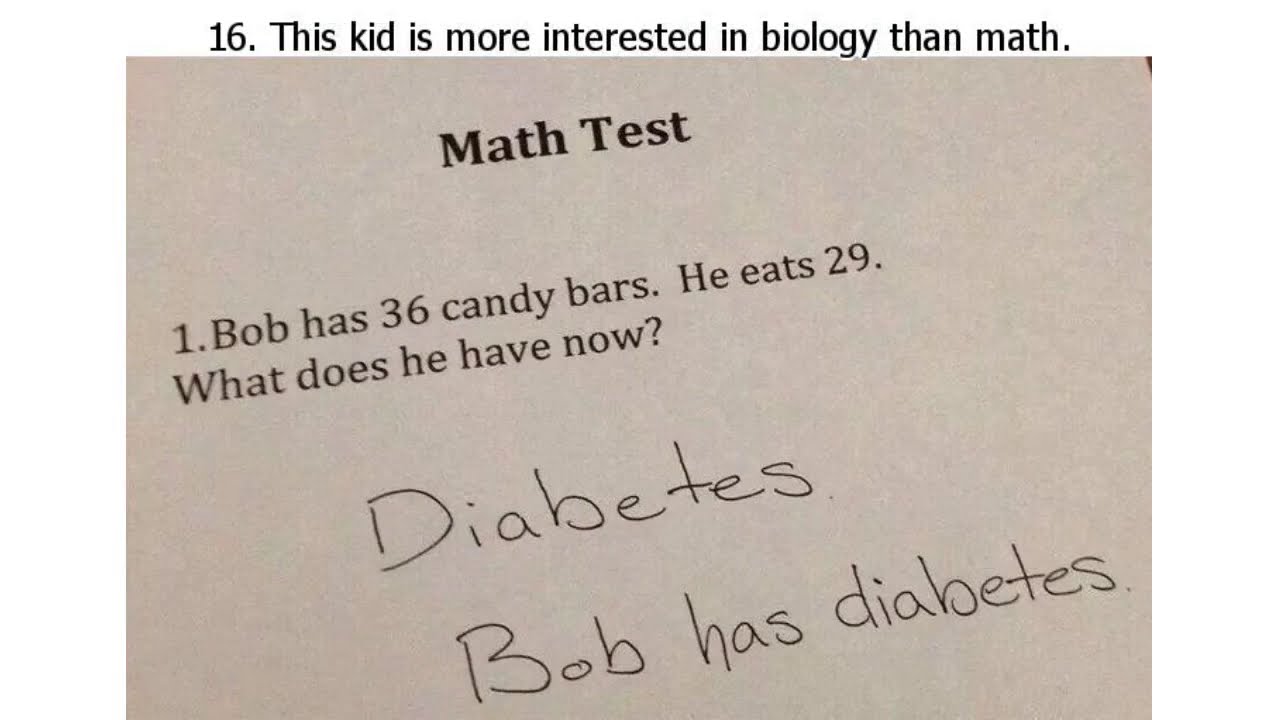The image is a meme featuring a close-up photograph of a math test question. On a typical white paper with a smooth surface, the test is titled "MATH TEST" in bold, dark letters. The question, marked as number one, reads: "Bob has 36 candy bars. He eats 29. What does he have now?" Humorously, the student's handwritten response underneath is: "Diabetes. Bob has diabetes." Adding to the humor, text above the image reads "16. This kid is more interested in biology than math," highlighting the student's unexpected yet funny answer.